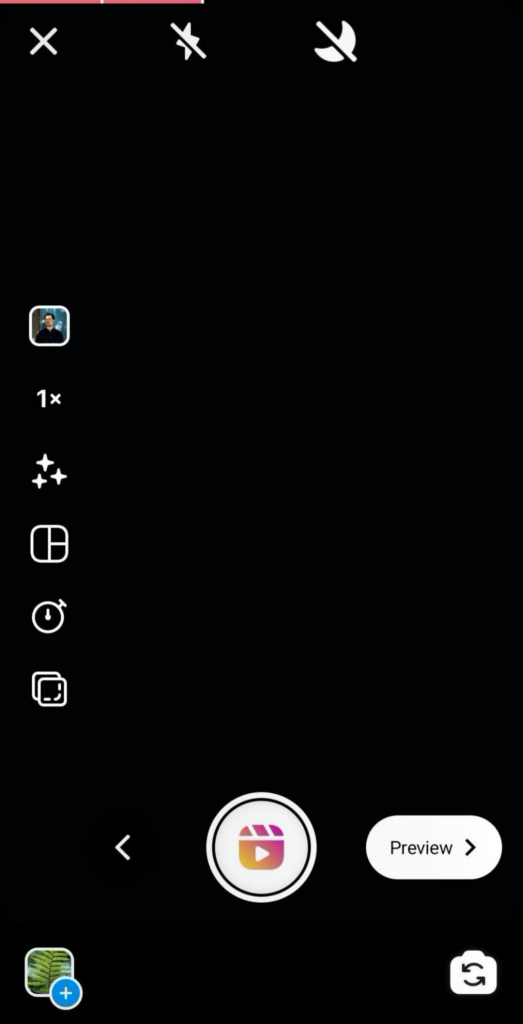The image is a square screenshot with a predominantly black background. Along the left-hand side, there is a vertical column featuring five icons in sequence. At the top, there's an icon resembling three stars. Beneath it, the second icon appears to represent a mouse with two buttons. The third icon in the series looks like a stopwatch. The fourth icon down the list depicts two computer screens superimposed on each other. At the very bottom of this column, a green icon with a plus sign is visible.

The majority of the upper section of the screenshot remains blank black space. About two-thirds down the image, a back button becomes visible. Adjacent to this, there is a white oval with a black outline containing a pink and orange icon displayed alongside a forward button. Across from this, another white oval is present with the label "Preview" and an arrow symbol. In the bottom right-hand corner, there are icons of a camera and symbols indicating the capability to move forward and backward.